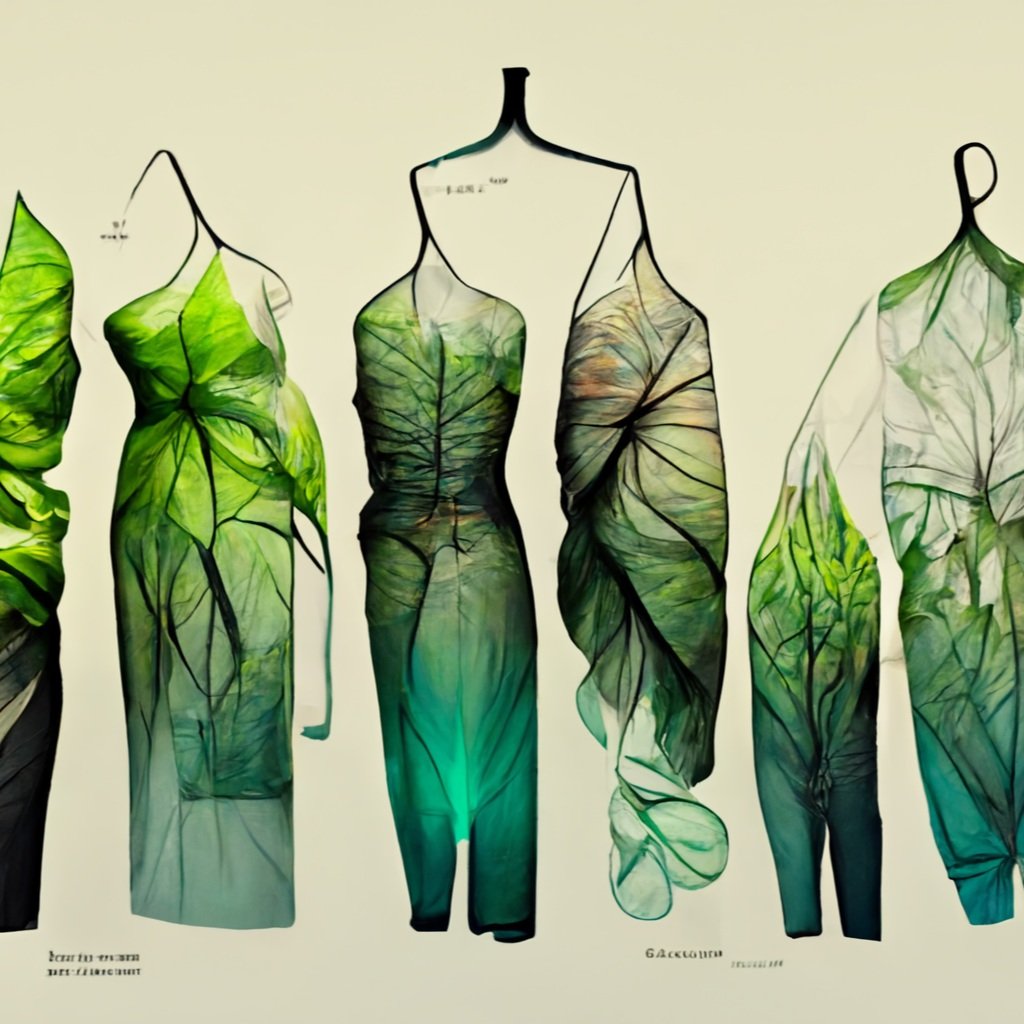This is a detailed and organic concept art of various clothing pieces inspired by leaves and natural elements. The scene features six outfits, arranged side by side against a clear cream-colored background, with two partially visible on the far left and right edges. The clothing items, including dresses, blouses, and possibly a jumpsuit, are designed with an earthy green palette that transitions from light green to dark green, almost turquoise. Branches at the top function as hangers, adorned with hooks to display the outfits. The garments mimic the appearance of leaves, complete with veins and different shades of green, creating a beautiful and artistic effect. At the bottom left and right corners, there is small, unreadable text, adding a subtle detail to this visually intriguing presentation.